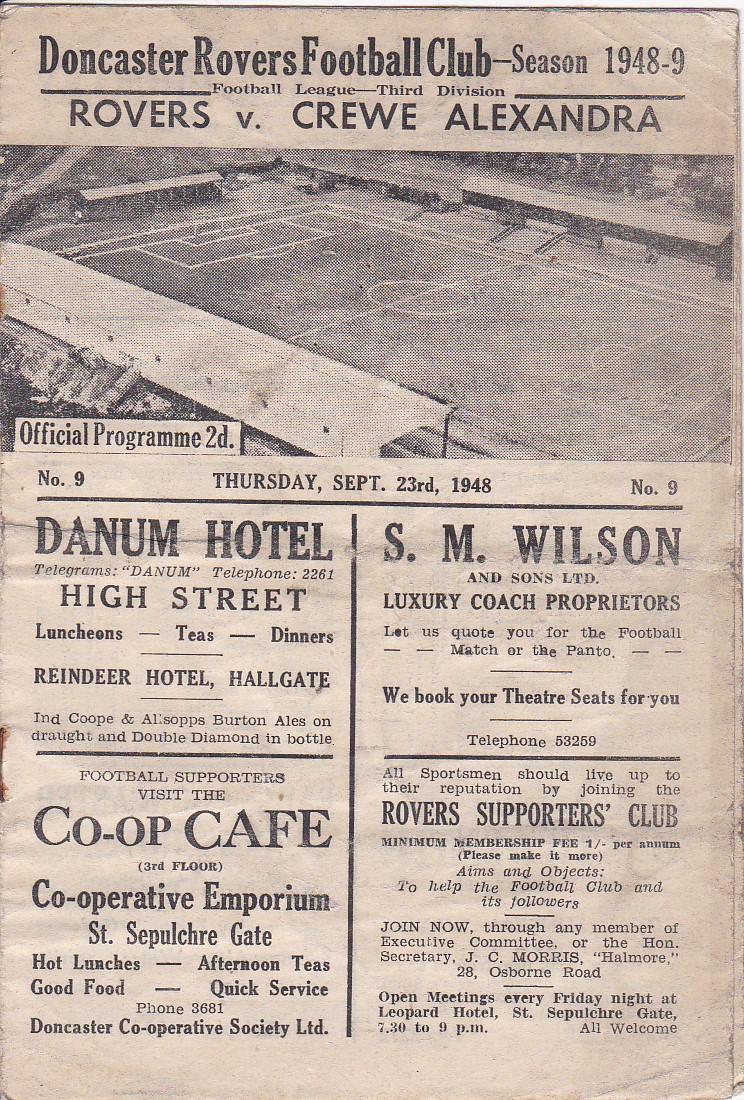The image depicts an official program for a football (soccer) match between Doncaster Rovers and Crewe Alexandra for the 1948-49 season in the Football League's 3rd Division. The program, dated Thursday, September 23rd, 1948, is in sepia tones, giving it an aged appearance. The top heading reads "Doncaster Rovers Football Club Season 1948-49, Rovers vs. Crewe Alexandra," with an associated black-and-white photograph of a soccer field surrounded by spectators. The front cover prominently states "Official Program 2D."

The bottom section of the program features several advertisements from local businesses:
- Danum Hotel on High Street offers luncheons, teas, and dinners.
- Reindeer Hotel located on Hallgate.
- Co-op Cafe and Cooperative Emporium on St. Sepulcher Gate, promoting hot lunches, good food, afternoon teas, and quick service, courtesy of the Doncaster Cooperative Society Limited.
- SM Wilson & Sons Limited, luxury coach proprietors, who also provide theater seat booking services.
- An invitation to join the Rovers Supporters Club with open meetings held every Friday night at the Leopard Hotel.

Overall, the detailed descriptions and array of advertisements reflect the community-oriented spirit of the 1940s football culture.